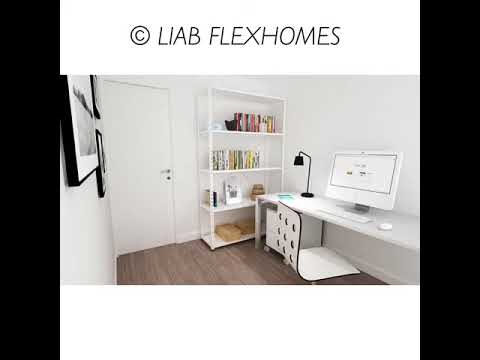This detailed photograph appears to be a well-styled bedroom, potentially used for a promotional image. The room is predominantly white, including the walls, bed, and shelves, which provides a clean and airy atmosphere. One of the walls is a large window divided into four sections by horizontal and vertical white frames, suggesting it may be a sliding glass door leading to a patio. 

The focal point of the room is a low, white bed with a white mattress situated against one of the walls. Above the bed, there are two white shelves. The top shelf holds a black and white photograph in a frame, while the lower shelf displays three round black objects, possibly vases or books. Adjacent to these shelves is a black and white painting depicting what looks like a Volkswagen bus, adding a touch of vintage charm to the space.

Directly opposite the bed, there is a brown desk accompanied by a matching brown chair with black armrests. On the desk sits a black laptop and a neatly stacked set of books. The room features a polished brown hardwood floor that adds warmth and contrast to the overall white theme. 

The image, bordered by black bars on the right and left sides, has a minimalistic yet inviting aesthetic, capturing a blend of modern and classic design elements. The careful placement of decor and furniture suggests this room is part of a promotional photograph for a company called Liab Flex Homes, indicated by the subtle branding above the main photograph. Overall, the photograph captures a serene and meticulously organized bedroom space.